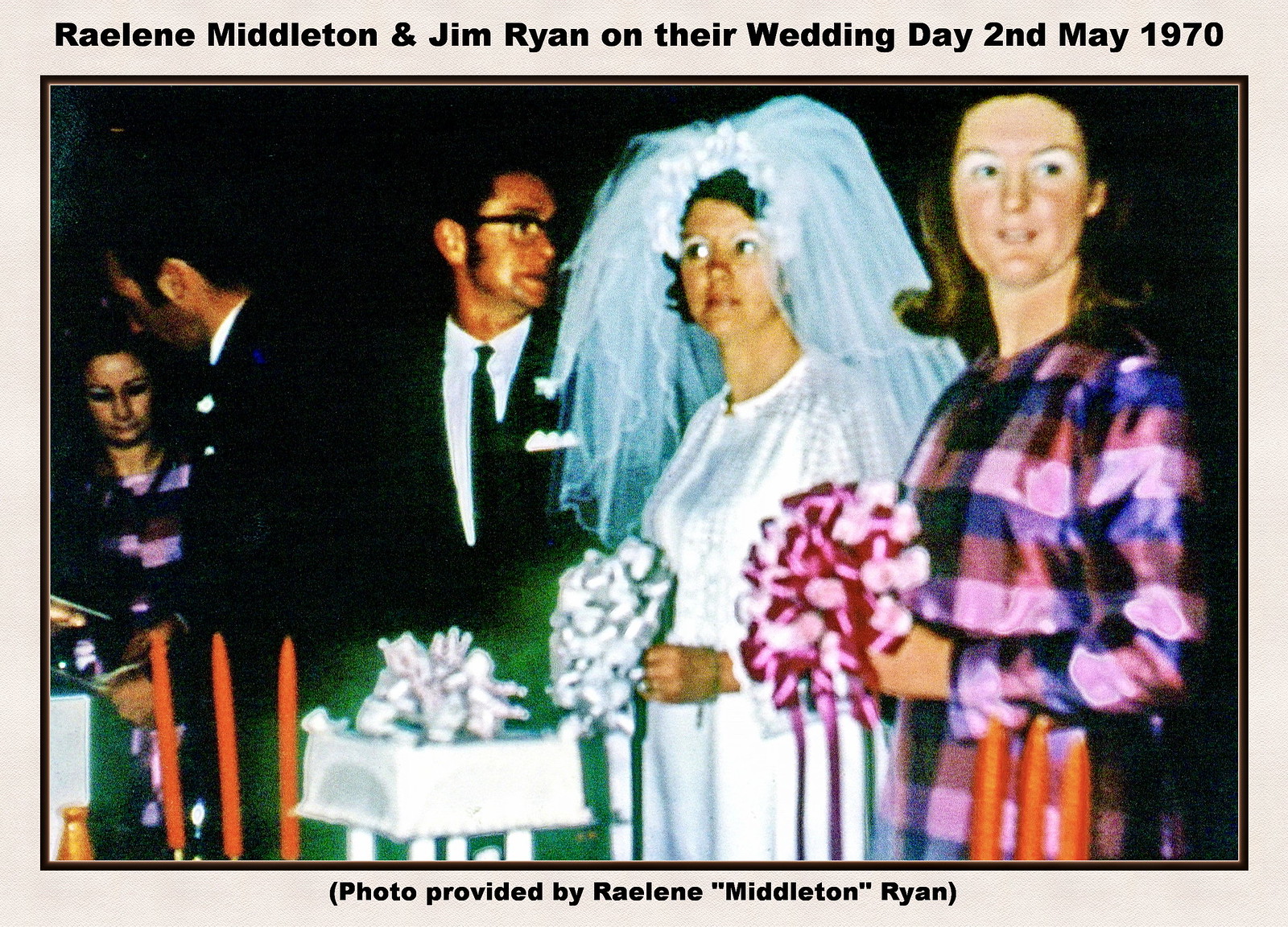This vintage photograph from May 2, 1970, showcases a wedding scene featuring five individuals. Central in the image is the bride, Raelene Middleton, adorned in a traditional white wedding dress with a light blue veil, and holding a silverish-blue bouquet. Beside her stands the groom, Jean Rian, dressed in a shirt, tie, and dark coat. Both are positioned in front of a wedding cake. To the left of the bride is a woman with dark black hair, dressed in a pink and purple flannel-like shirt, holding a red and white bouquet. On the far right, another woman holds flowers. The image, which appears grainy and somewhat faded, has a light gray border with text. The top of the border reads "Raelene Middleton and Jean Rian on their wedding day 2 May 1970," while the bottom notes, "(photo provided by Raelene Middleton Rian)." In the background, additional guests are seen engaging in conversation, adding to the celebratory ambiance.